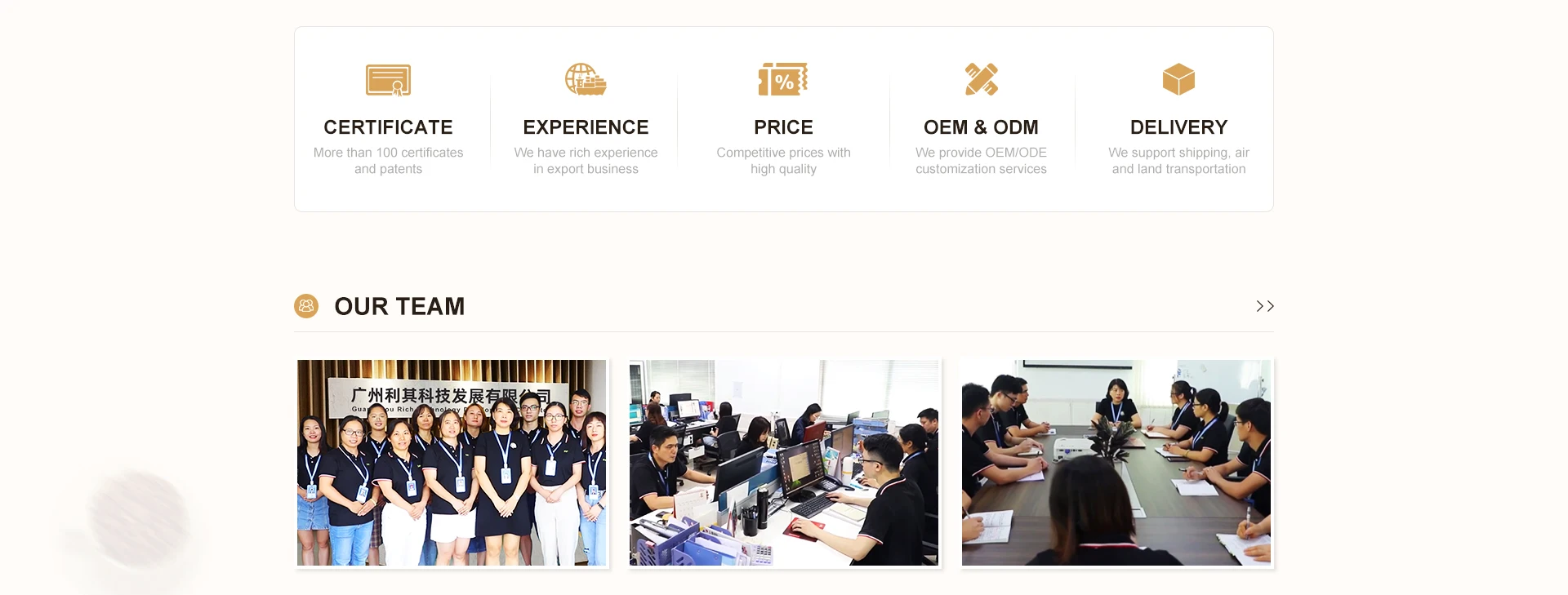This personal website of an unnamed company features a clean design with a beige background. At the top of the page, there are five distinct options illustrated with icons and detailed scope of services. 

1. **Certificates:** Represented by a gold certificate icon, it highlights that the company holds more than 100 certificates and patents.
2. **Experience:** Marked by a relevant icon, this section emphasizes the company's extensive experience in the export business.
3. **Price:** Accompanied by an icon, this box assures customers of competitive prices without compromising on high quality.
4. **OEM & ODM:** Displayed in bold black capital letters with a grey subtext, this section indicates that the company offers OEM and ODM customer services.
5. **Delivery:** Illustrated with a distinct icon, it underscores the company's support for shipping via air, land, and sea transportation.

Beneath these options is a section titled "Our Team," showcased with an icon in capital letters. Below this title, three photographs convey the team’s dynamics: 
- A group photo of the team standing together,
- An image of team members diligently working at their computers,
- A shot of the team engaged in a business meeting around a desk.

Each element is meticulously crafted to present the company’s credentials and capabilities in a professional and comprehensive manner.